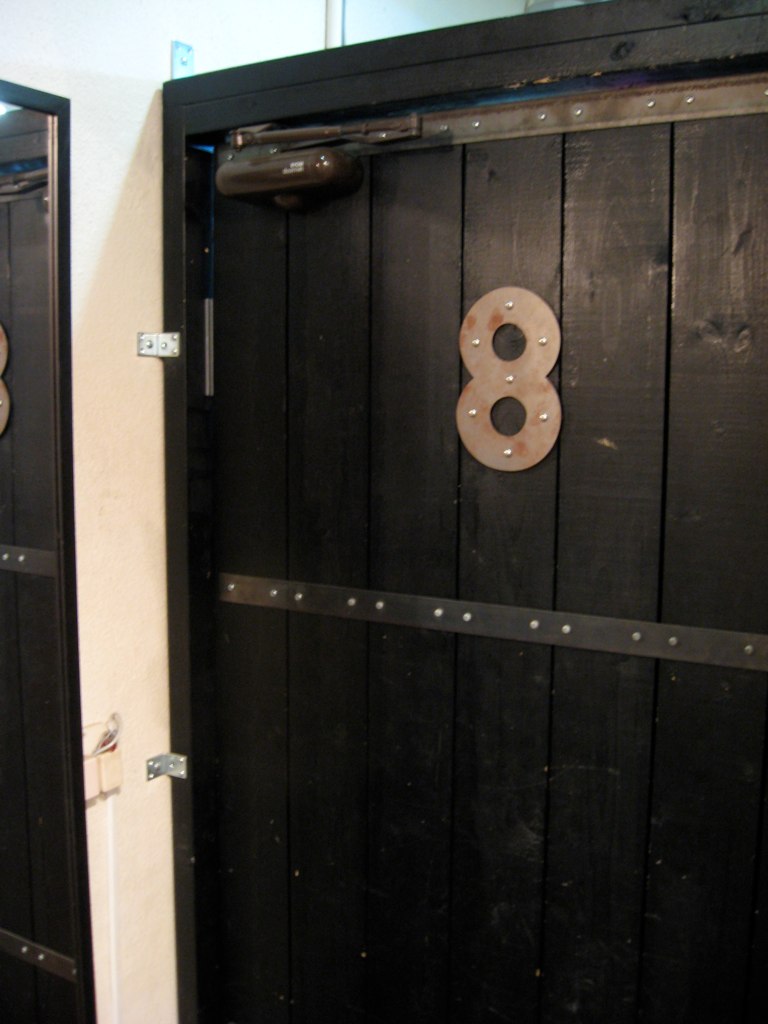The image portrays a dark, almost black, wooden door with vertical panels and adorned with meticulously placed silver rivets. Centrally mounted on one of the panels is a metal number 8, secured with similar silver rivets. A horizontal metal strap runs across the middle of the door, featuring rivets organized in groups of two, spaced equally throughout its length. To the left of the door, partially cut off, is a mirror reflecting part of the door and the number 8. The adjacent wall, between the door and the mirror, is painted an off-white color. The door is equipped with a fire escape closure device at the back, which ensures it closes automatically. The door also has several silver-toned hinges attaching it to the frame, which is dark brown and holds the structure securely in place.